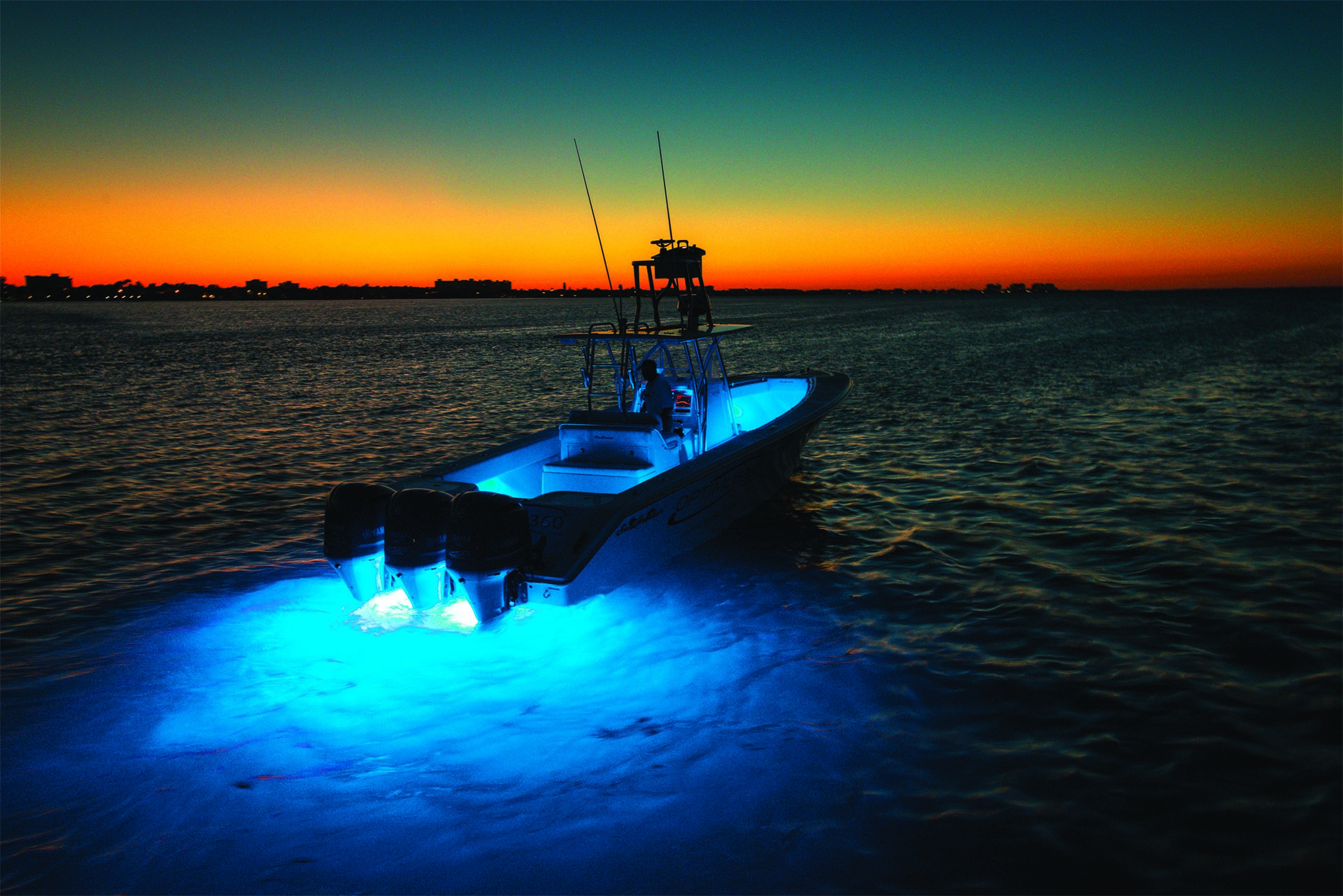This captivating image, enhanced with CGI effects or photo filters for dramatic lighting, captures a scene at dusk with vibrant, exaggerated colors. The primary focus is a speedboat, approximately 16 to 18 feet long, equipped for fishing with visible fishing poles and a seated driver. The boat is powered by three outboard engines and features a small platform at the stern. As the boat moves away from the shore, it leaves behind a striking deep blue wake, likely illuminated by blue neon lights installed at the back. These lights also cast a glow inside the open bow boat, creating a turquoise and blue luminescence that contrasts the rippled, dark water. On the distant horizon, a thin, shadowy strip of land and scattered silhouettes of buildings can be seen against the backdrop of a vivid orange sunset bleeding into a darkening sky. The captivating, slightly surreal hues of the scene highlight the beauty of the moment, blending natural elements with artificial enhancements.